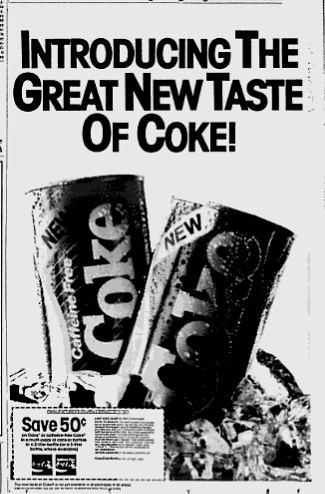This vintage black-and-white magazine advertisement for Coca-Cola measures approximately 2 inches wide by 3 inches high and features a light gray background with black text. Dominating the top third of the page is a bold, large-font headline reading, "Introducing the Great New Taste of Coke." Below this, two aluminum cans of Coca-Cola are depicted nestled in a pile of ice. The can on the left is labeled "Caffeine-Free Coke" with an upward diagonal banner that says "New," while the can on the right simply reads "Coke" with a similar "New" banner. Along the left-hand side of the ad is a small vertical borderline. In the lower left-hand corner, there is a horizontal rectangle with a dotted black line around it, designed to look like a coupon, featuring the text "Save 50 Cents" and an image of the Coca-Cola logo beneath it. This advertisement evokes a sense of nostalgia with its simple, yet eye-catching design and promotional offer.